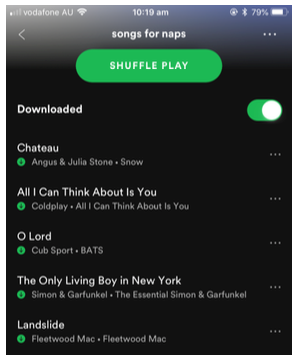In the detailed image, we see a Spotify playlist open on a device screen. At the very top, the notification bar displays Vodafone AU, alongside the Wi-Fi icon, indicating active internet connectivity. The screen shows it's 10:19 AM, with the Bluetooth icon next to the time, followed by a battery indicator showing 79%.

Beneath the notification bar, there is a navigation bar with a left arrow, suggesting a back function. Centered prominently is the playlist name "Songs for Naps," accompanied by a green "Shuffle Play" button encouraging random song play.

Below this, a download status indicated by the text "Downloaded" accompanied by a green toggle switch shows that the playlist is actively downloaded.

The playlist starts with "Chateau" by Angus & Julia Stone, from their album "Snow," with a green download arrow next to the song, signaling it's downloaded. The following song is "All I Can Think About Is You" by Coldplay. The third track listed is "Oh Lord" by Cup Sport and B.A.T.S. Further down, "The Only Living Boy in New York" by Simon & Garfunkel, from the album 'Essential Simon & Garfunkel,' is displayed. The final song in the visible list is "Landslide" by Fleetwood Mac.

The overall interface features a sleek, all-black background typical of Spotify's aesthetic, emphasizing the playlist details and controls.